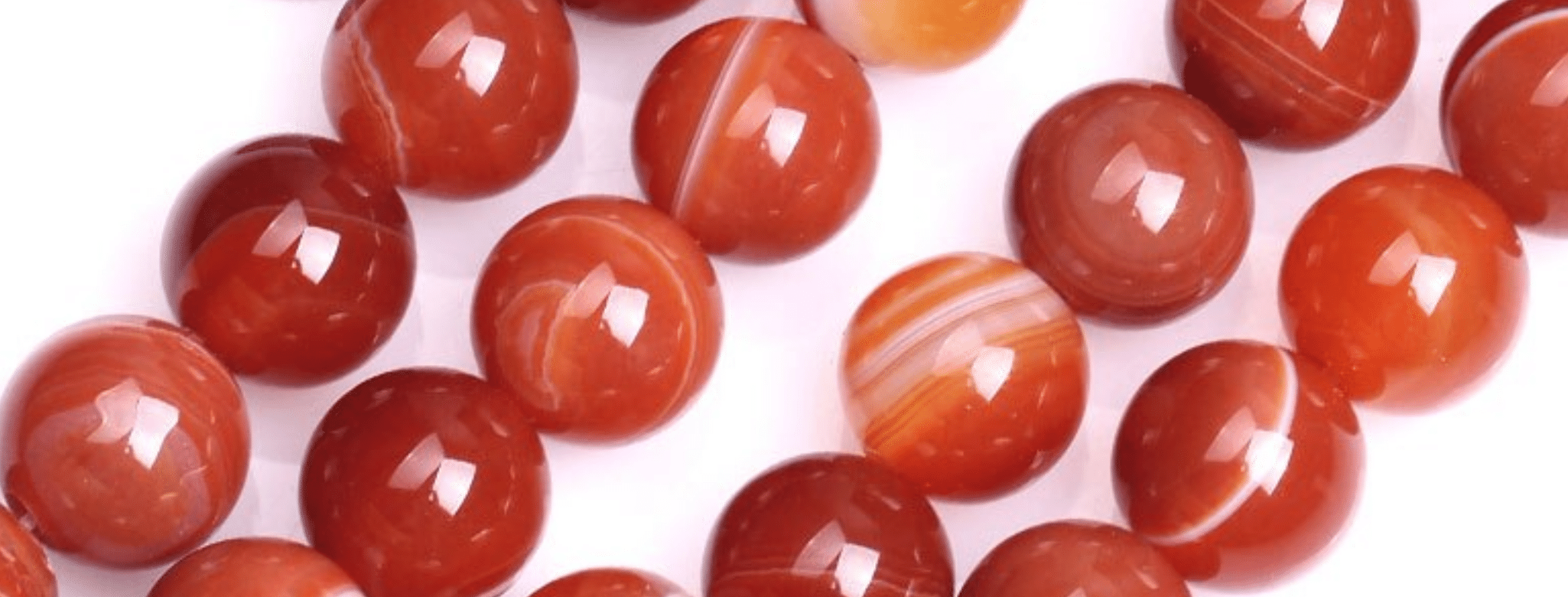This indoor photo features a close-up display of marbles arranged on a pristine white background, likely intended for an online sale. The scene includes four columns of marbles that run diagonally from the lower left to the upper right, contributing to an artistic layout. Each column contains marbles varying slightly in design but sharing a common color palette of reddish terracotta hues, complemented by streaks of white. The marbles—approximately 16 to 20 in total—exhibit vivid reflections due to the ambient light, enhancing their glossy appearance. This thoughtfully arranged setting, reminiscent of artistic or commercial photography, emphasizes both their uniformity and individual nuances.